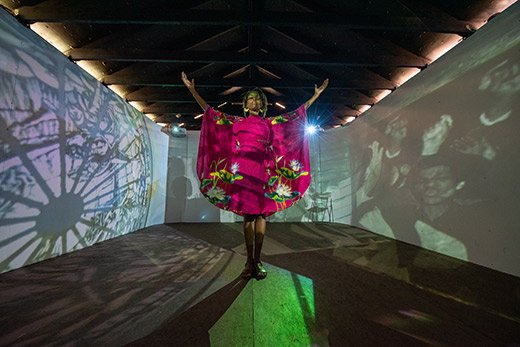In this animated image, a Black woman stands centered in a room with her arms raised to her sides. She is adorned in an elaborate pink dress decorated with white flowers and green lily pads, which extends just above her knees and slightly past her elbows. The background reveals a room with a wooden rafter ceiling and gray walls adorned with different projected images. To her right, a projector screen displays a scene of people, while another screen on the left may show figures engaged in protest or a clock. Light filters into the room from just beneath the rafters, casting reflections on the wooden floor. The floor itself appears intriguingly painted with green and blue hues, creating the illusion of an opening. The setting suggests a presentation or a display, possibly held in a gallery-like space.